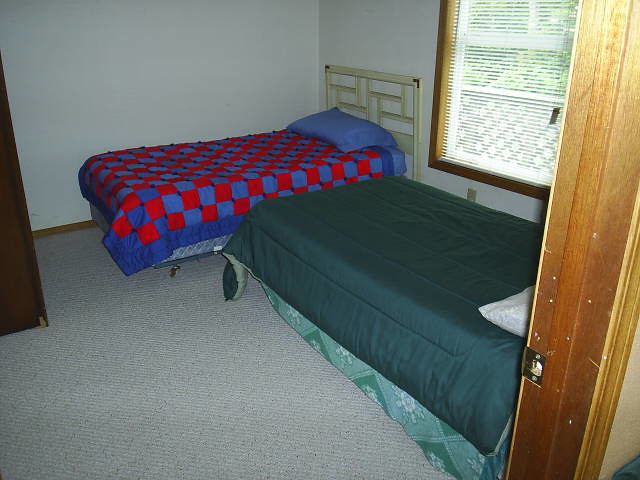The photo captures a detailed view of a bedroom with light blue walls and a gray carpet. In the upper right corner, there's a window with white mini blinds, through which a white fence and some trees are faintly visible. The bedroom features two single beds positioned perpendicular to each other. 

One bed, located in the bottom right, is positioned diagonally from southeast to southwest. It has a dark green blanket with a lighter green pattern, which includes white and slightly darker green designs, such as white flowers and triangles. A white pillow lies on top, near the bottom right corner of the bed. 

The second bed is in the top middle of the room and features a checkered blanket with blue and red squares, complemented by a dark blue sheet and pillow. 

To the far right, the wooden door frame of the entrance to the bedroom is visible. Near the left-hand side of the image, there appears to be part of a door or some brown-colored object. There is also a tan wall on the far right, adjacent to the door jamb. Something blue is visible in the lower right corner, adding a bit of color diversity to the scene.